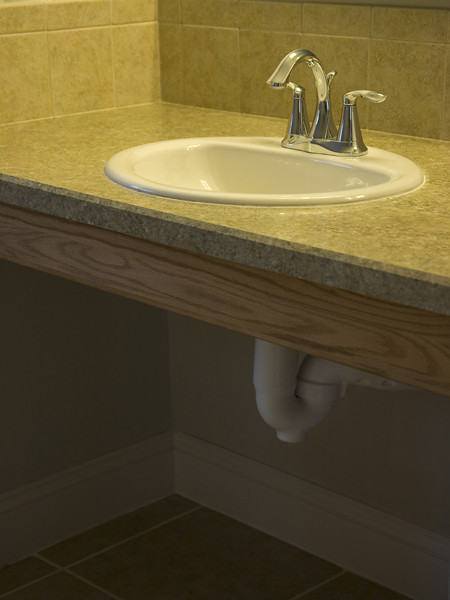The image depicts a bathroom interior focused on a sink area. The surrounding wall tiles are predominantly gray with subtle yellow undertones, accentuated by linear patterns running through them. The countertop is made of white granite, featuring speckles that add depth and texture to its surface. The sink, crafted from white porcelain, is adorned with sleek silver handles and a matching faucet. The polished faucet casts a slight reflection on the porcelain basin, which appears to be illuminated by overhead lights. 

The front of the sink stand is made of wood, showcasing distinctive wood grains. Underneath the sink, the exposed PVC pipes are visible, extending downward before curving up and disappearing into the wall. The lower portion of the image is relatively dim, revealing black floor tiles and white trimming along the base of the wall. The background maintains a consistent gray theme, complementing the bathroom's overall color scheme. Notably, the wood on the edge of the sink stand features a circular graining pattern, adding an intricate detail to the design.